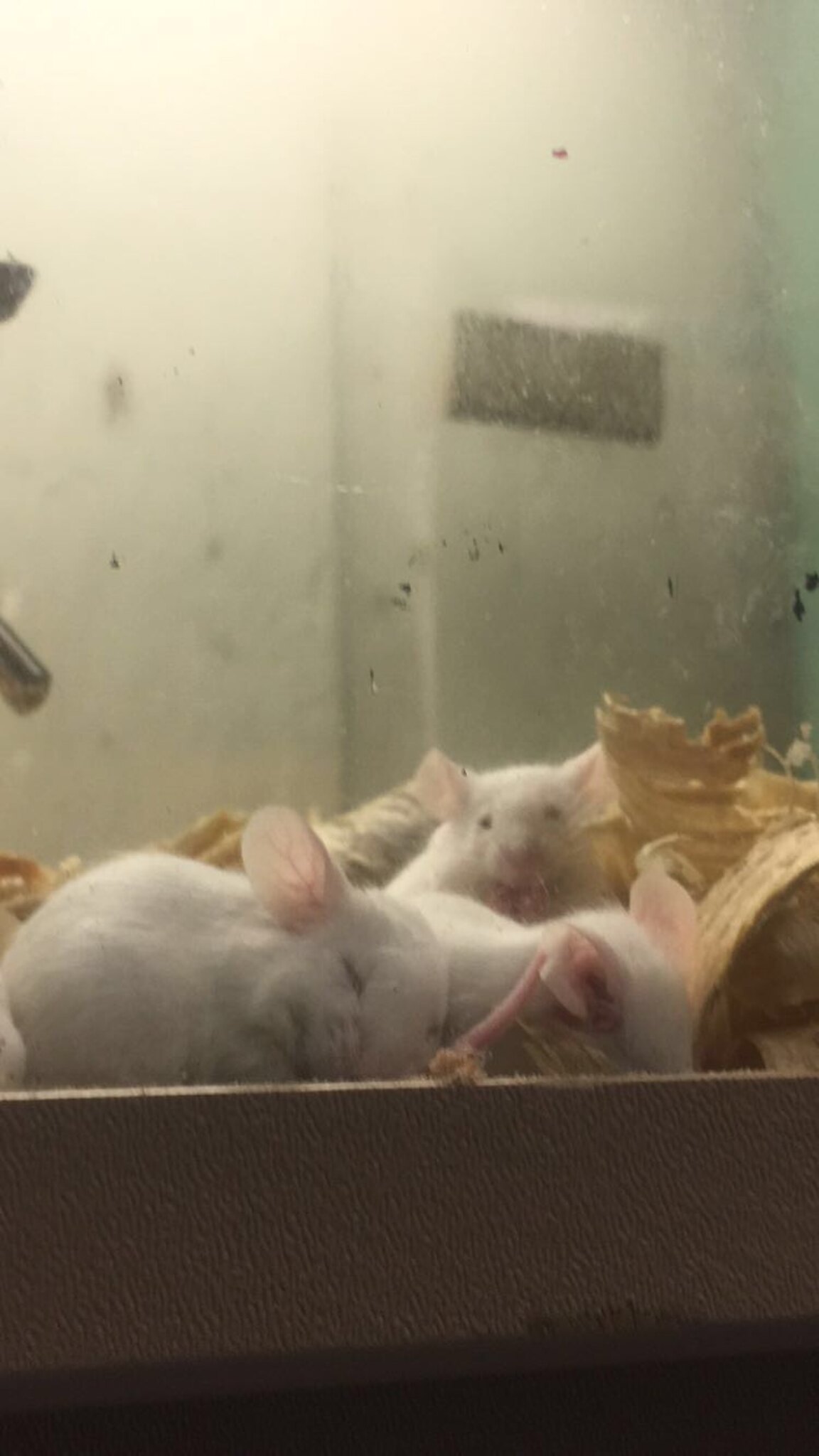The image depicts a cage with a concrete stone bottom, filled with beige shavings or wood chips. Inside the cage, there are three white mice with pink ears, noses, and limbs. Two of the mice are lying down with their eyes closed, indicating they are sleeping, while the third mouse in the back is awake, sitting upright, and staring directly at the viewer. The background features a white wall with a brown or black rectangular object on it. Additionally, silver drinking cylinders are visible on the upper left side of the cage, likely for dispensing water. The enclosure appears to be glass, evidenced by the slightly cloudy or fingerprinted surface reflecting an overhead light, suggesting a somewhat unclear view of the surroundings.